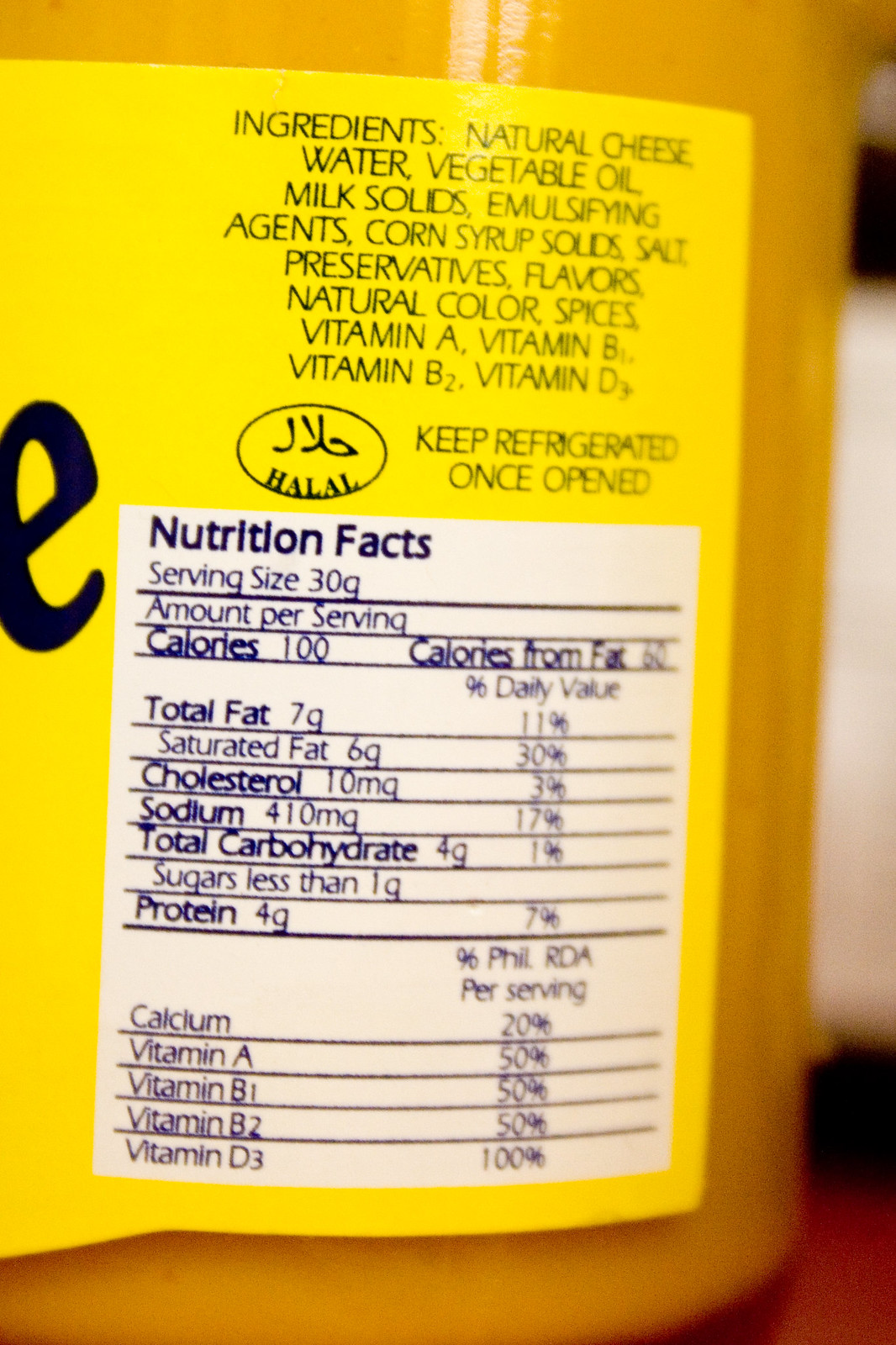The image displays a yellow-gold plastic container likely holding a cheese product. Prominently featured on the container is a bright yellow label with a detailed ingredients list and nutritional information. The label includes black text listing ingredients such as natural cheese, water, vegetable oil, milk solids, emulsifying agents, corn syrup solids, salt, preservatives, flavors, natural color, spices, vitamin A, vitamin B1, vitamin B2, and vitamin D3. The label also advises keeping the product refrigerated once opened and includes a halal symbol in an oval shape. Below the ingredient list, there's a white box with black text presenting the nutritional facts: serving size 30 grams, 100 calories per serving (60 calories from fat), 7 grams of total fat (11% DV), 6 grams of saturated fat, 4 grams of carbohydrates, 4 grams of protein, and percentages for calcium and vitamins A, B1, B2, and D3. The container appears to be situated on a surface with a hint of red visible in the bottom right corner.